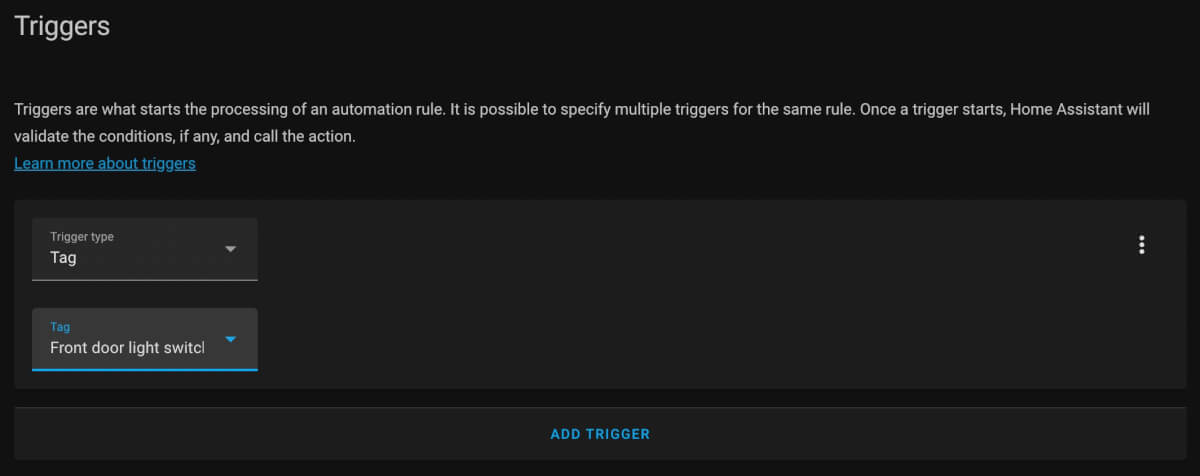This screenshot captures a section of an auction page with a dark theme, featuring a black or dark gray background. In the upper left corner, white text prominently displays the word "Triggers," accompanied by explanatory text in smaller font: "Triggers are what start the processing of an automation rule. It is possible to specify multiple triggers for the same rule. Once a trigger starts, Home Assistant will validate the conditions, if any, and call the action."

Beneath this descriptive text, a blue hyperlink labeled "Learn more about triggers" is visible, inviting users to delve deeper into the topic. The main focus of the screenshot is a slightly lighter gray box showcasing several options. The first option includes a drop-down menu labeled "Trigger type" followed by "Tag," with a small arrow indicating the presence of a selectable menu.

Underneath this, another slightly lighter box is shown with "Tag" in blue at the top, and "Front Door Light Switch" in white text. This is truncated, with a blue drop-down arrow and a blue underline hinting at a modified or active setting. In the top right corner of this box, three vertical dots likely represent additional settings or menu options.

Below this, a separate box of the same color features blue text in the center, stating "Add Trigger," suggesting the functionality to introduce additional triggers. Overall, the screenshot appears to be from the settings section of Home Assistant, where users can define various triggers to automate their smart home rules.